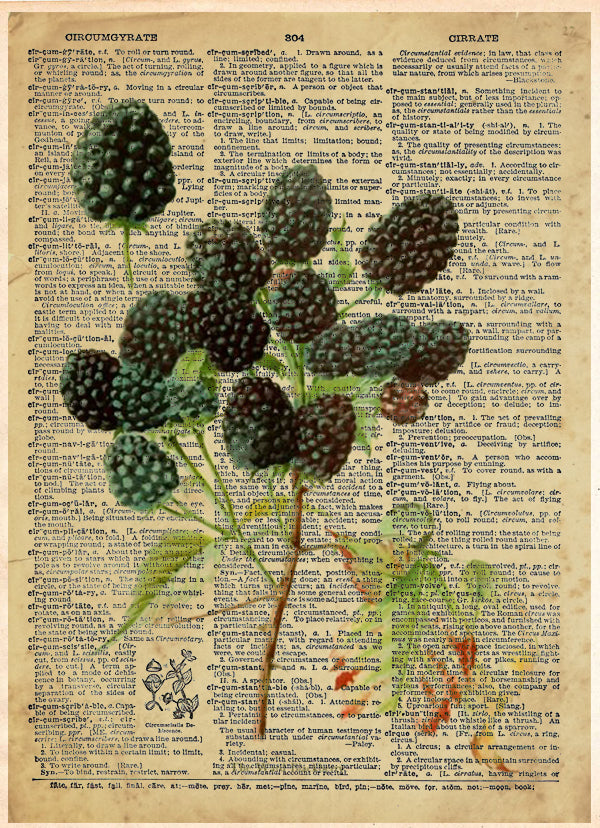The image depicts a branch of blackberries meticulously arranged against the backdrop of an aged, yellowed dictionary page, featuring three columns of densely packed black text. The blackberries exhibit a striking black-purplish hue, appearing almost three-dimensional. Notably, the berries remain pristine and intact, as if unaffected by the pressing process, suggesting an artificial composition. The stem of the plant rises from the bottom of the page, adorned with leaves that intertwine among the berries, forming a bouquet-like arrangement at the top. Additional colorful elements, in hues of red, green, yellow, and burnt orange, appear as blobs in the lower right corner of the page, contributing to the visual complexity. Three-quarters down the first column on the left, a small hand-drawn image adds a touch of intricacy. Despite the visual realism, the clean and unsullied appearance of the berries and lack of bleed-through onto the paper imply that the scene is a crafted illusion rather than a true botanical pressing.